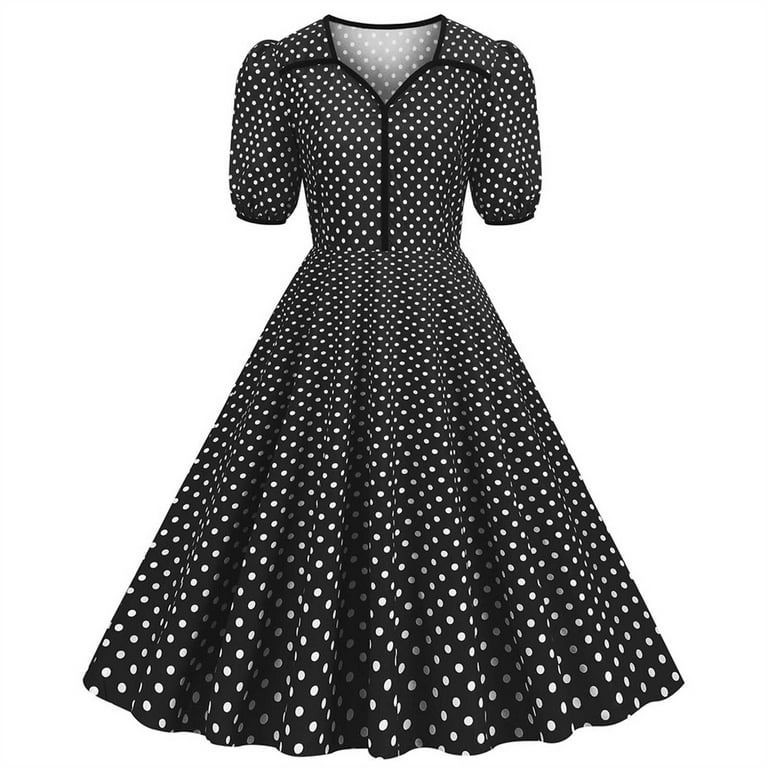The image features a vintage-style black dress adorned with white polka dots, displayed against a white background. The dress is presented in a manner that shows both the front and the inside back near the neckline. It has long, slightly puffy sleeves that extend to the elbows. The polka dots vary in size, starting smaller at the blouse section, becoming even smaller at the waist, and larger and more spaced apart toward the bottom. A distinctive black line runs from the waist up to the top and fans out to both shoulders. The fitted waist flares out elegantly in ripples, creating a flowing, blossomy skirt that likely descends to the shins. Crafted without zippers or buttons, it's essential to ensure a proper fit due to its fixed size. Overall, it's a pretty, detailed dress evocative of 1950s fashion.